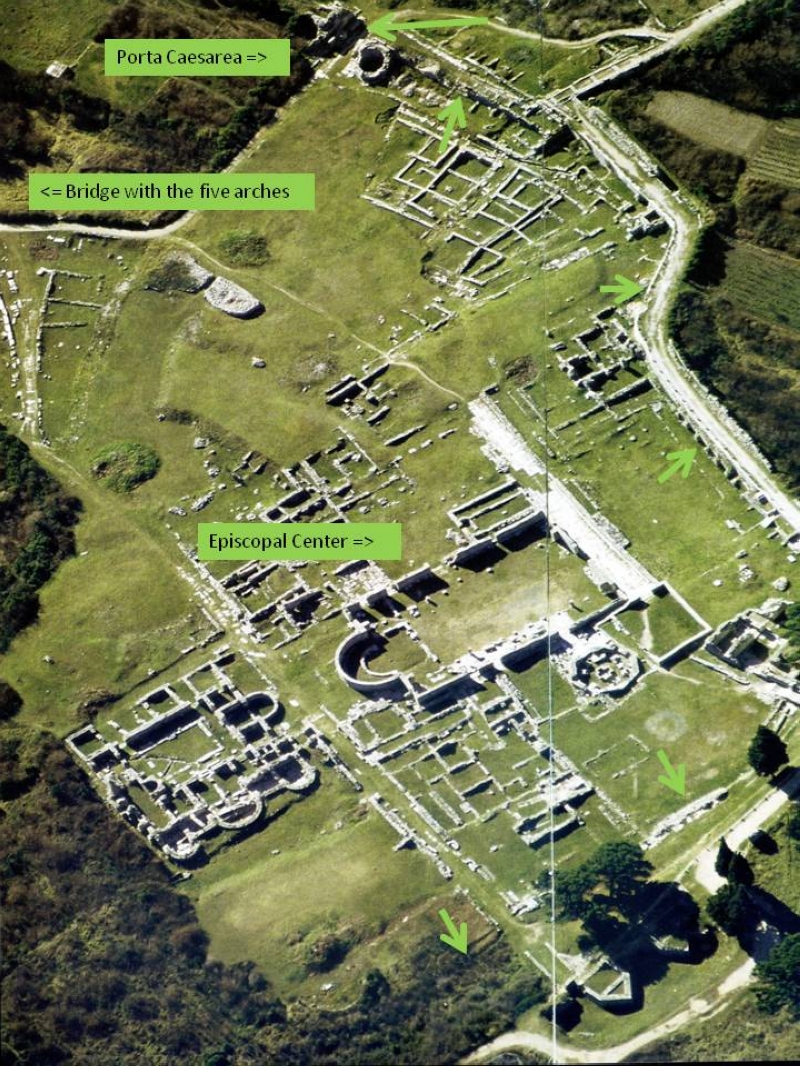The image appears to be an aerial photograph, likely from a textbook, showing a verdant landscape interspersed with historical ruins and detailed with several labels. Dominating the scene, the lush greens of farm fields and wooded areas frame the main features. In the upper section, an arrow points to a large excavation site marked as "Puerto Quesarey." Below and slightly leftward, another label identifies the "Bridge with the Five Arches," though the bridge itself isn't clearly visible. The central part of the map highlights the "Episcopal Center," also indicated with a prominent arrow. Smaller arrows scattered across the image point toward various roads and additional elements within the expansive, green expanse. The landscape, dotted with ruins and enclosed by evergreens, presents a maze-like appearance, suggesting it may be a historically significant area.